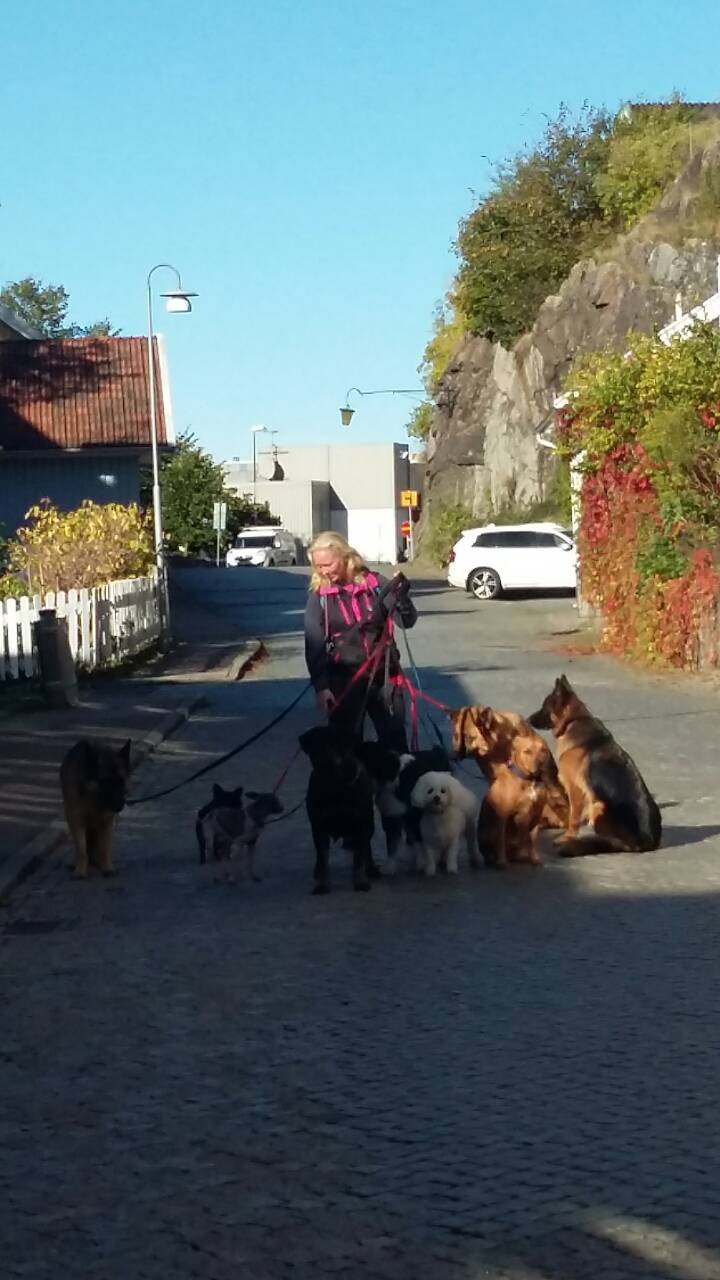In the photo, a professional dog walker is captured managing an impressive group of 12 dogs on a cobblestone alleyway. The scene is set under a bright blue sky, though the sun casts a shadow partially over her, indicating the sun is positioned behind her. The cobblestone path, dark gray or black, adds texture to the scene, and to the right, there is a living wall covered in vines and small bushes. On the left, a white picket fence lines a small sidewalk, leading to a house. 

The dog walker is a woman with blonde hair, dressed in a black jumpsuit with pink suspenders. She expertly holds the leads of a diverse mix of dogs: large breeds like two German Shepherds and a Pit Bull, medium-sized ones like a poodle, and smaller breeds including a Chihuahua. They all appear well-behaved, either sitting or walking in sync. A white SUV, resembling a Toyota, is parked behind her, with rock cliffs and buildings in the backdrop, hinting at an urban setting enveloped in nature. The woman is looking down at the dogs, ensuring they are all under control as she walks along this picturesque, serene alleyway.